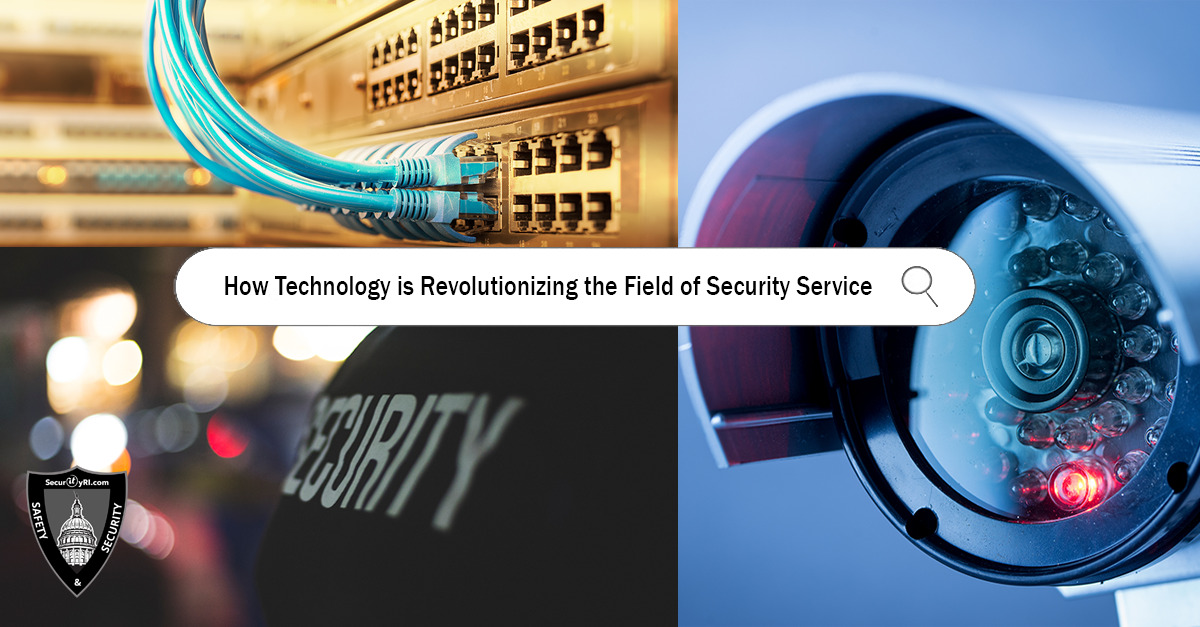This composite image, likely an advertisement, is split into two distinct sections showcasing advancements in security technology. On the left, a detailed close-up reveals a security system setup featuring multiple blue Ethernet cables connecting to a gold-colored router or modem. Below this, the black t-shirt of an individual, with the word "SECURITY" boldly printed across the chest, signals their role in the security field. In the lower left corner, a badge-like emblem contains the words "SAFETY" and "SECURITY" flanking an image reminiscent of the U.S. Capitol dome, with an obscure website at the bottom. The blurred background includes various lights, creating an impression of a cityscape. On the right side, a sharp, close-up image showcases a modern security camera with a prominent lens and a small, distinct red dot. The background here transitions into a hazel blue color, emphasizing the advanced and sleek nature of the surveillance equipment.